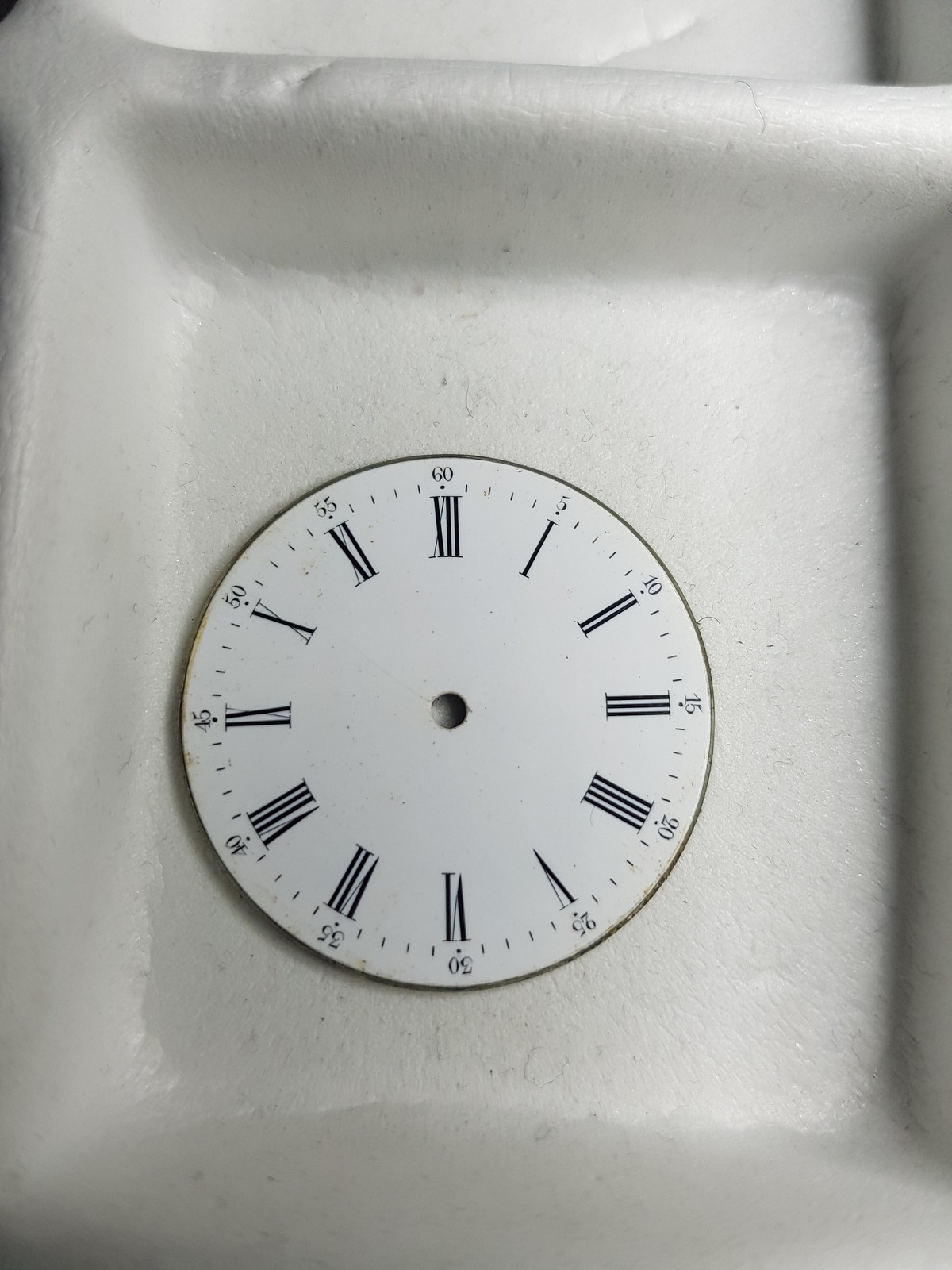This image features a pristine white clock face, prominently positioned within a shallow, rectangular basin. The clock face is notably devoid of hands, showcasing an empty central hole. The design includes dual numerical graduations; the inner ring is marked with Roman numerals from I to XII, while the outer ring is detailed with Arabic numerals in increments of five, spanning from 5 to 60. The simplicity of the dish and the clarity of the markings on the clock face emphasize its minimalist aesthetic.